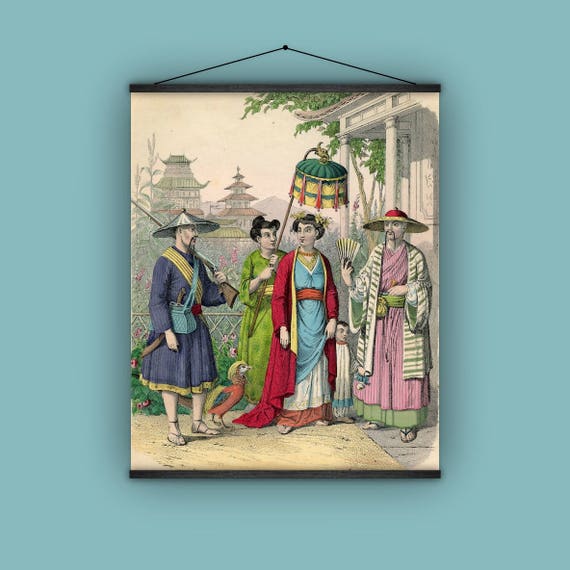The image is a square photograph of a wall painted in a serene shade of light teal. Centered at the top of the wall, a tapestry-style print is meticulously hung from a nail by two delicate black threads, further secured by a substantial black wooden band at both the top and bottom edges. The tapestry itself features a tranquil cream-colored sky backdrop and depicts a group of four Asian individuals, two men and two women, positioned in the foreground with intricate detail.

To the left, the first man, identifiable by his tin hat and open-toed sandals, carries a gun slung over his left shoulder and directs his gaze toward the center. Beside him, a woman dressed in a light green dress holds a green-and-yellow umbrella, shading the second woman, who stands central in the frame. This central woman is elaborately dressed in layers: a blue dress adorned with a red belt and a yellow-trimmed red robe, which drapes over a white skirt, under which is another red skirt; she wears no shoes and has a necklace around her neck.

To the right, another man stands out with his striking red wide-brimmed hat accented with yellow. He wears a pink robe underneath a green dress, topped with a green-and-white robe, and blue sandals. In his right hand, he holds a fan, and his long, thin mustache completes his distinguished appearance.

The background of the tapestry reveals a city scene with traditional Asian architecture, including stone buildings with columns and tiered, flared roofs. A colorful bird, with a red body and blue-and-yellow feathers, also stands near the group, adding to the tapestry's rich narrative and intricate detail.